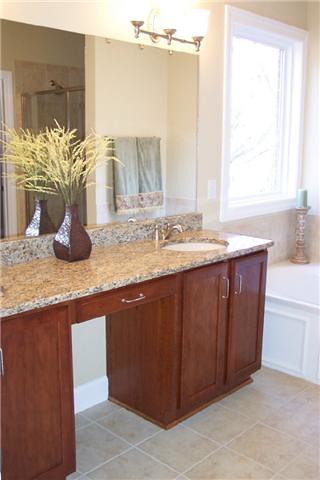Image Caption: 

This detailed bathroom scene features tan walls and a sleek silver light fixture equipped with three illuminated bulbs. Dominating the room is a large rectangular mirror that vividly reflects various elements of the space. Within the mirror, green bath towels are seen hanging on the wall, complemented by a mix of tan and grey tiles that line the floor and wall. A glass shower door can also be observed in the reflection.

The countertop below the mirror is adorned with a brownish-gray marble surface, hosting a stylish brown vase filled with an arrangement of green and yellow foliage. A pristine white sink, complete with a shiny silver faucet, is centrally located on the countertop. Brown cabinetry, including a slender drawer in the middle and dual cabinet doors with silver handles, sits neatly beneath the sink. Part of an additional door is visible, offering a glimpse into a window and bathtub area beyond it.